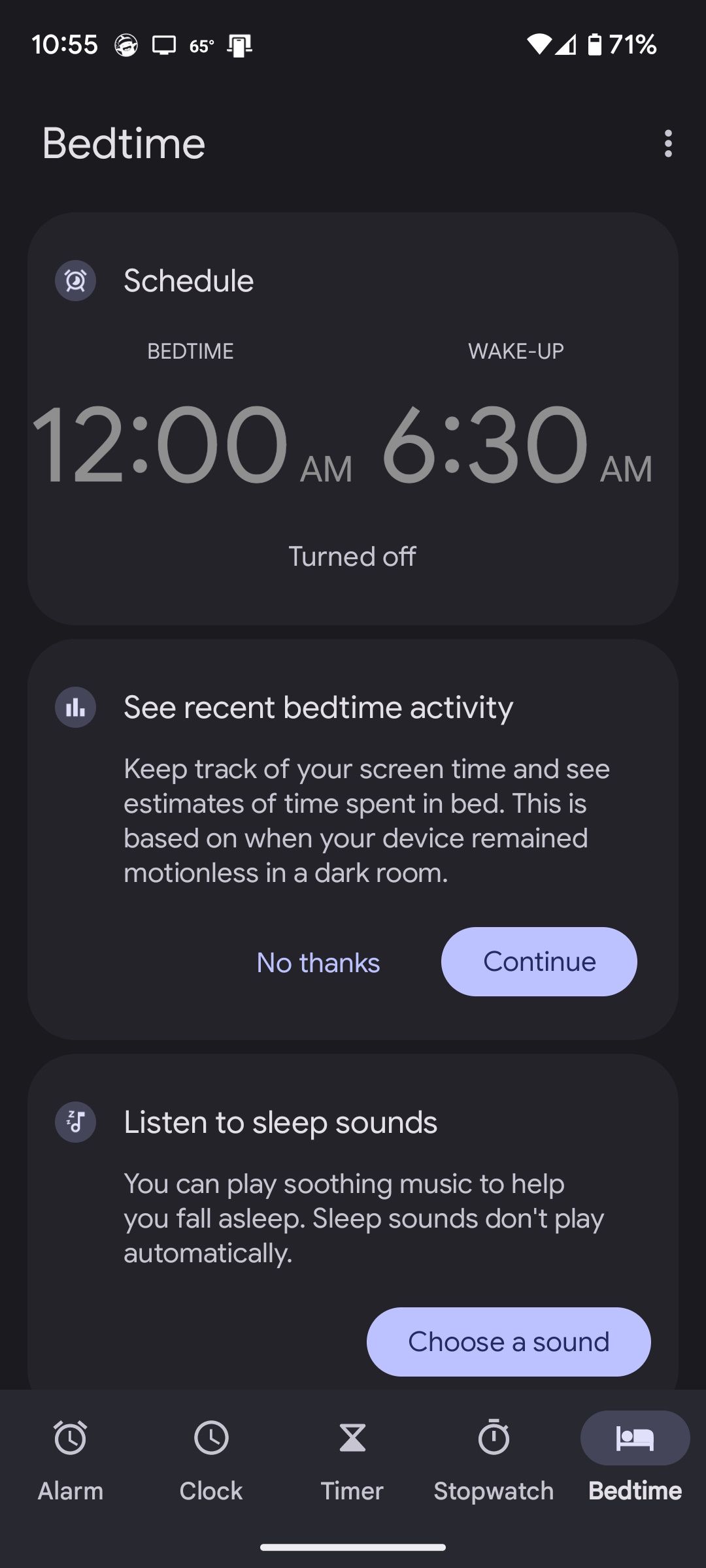The image depicts an iPhone screen displaying the Bedtime feature within the Clock app. The iPhone battery is at 71% charge, and the time shown at the top left corner is 10:55. Various white icons are visible in the status bar.

At the top of the screen, a section is labeled "Bedtime." Beneath this heading is the text "Schedule," accompanied by an icon of a clock. Below, the schedule specifics are outlined, indicating the bedtime is set for 12:00 a.m. and wake-up time is set for 6:30 a.m. Currently, the schedule is turned off.

The screen also offers the option to "See Recent Bedtime Activity," where users can keep track of their screen time and view estimates of time spent in bed, based on when the device remained motionless in a dark room. Users can choose "No Thanks" or "Continue," with the latter written in a periwinkle color.

Further options include "Listen to Sleep Sounds," which offers the ability to play soothing music to help with falling asleep. It notes that sleep sounds do not play automatically and provides the option to "Choose a Sound" within a purple periwinkle-colored circular button.

At the bottom, there is a navigation bar for the Clock app featuring the following icons: an alarm clock for the Alarm section, a traditional clock face for the Clock section, an hourglass for the Timer section, a stopwatch for the Stopwatch section, and a bed for the Bedtime section. A thin white line spans the bottom of the screen, completing the layout.